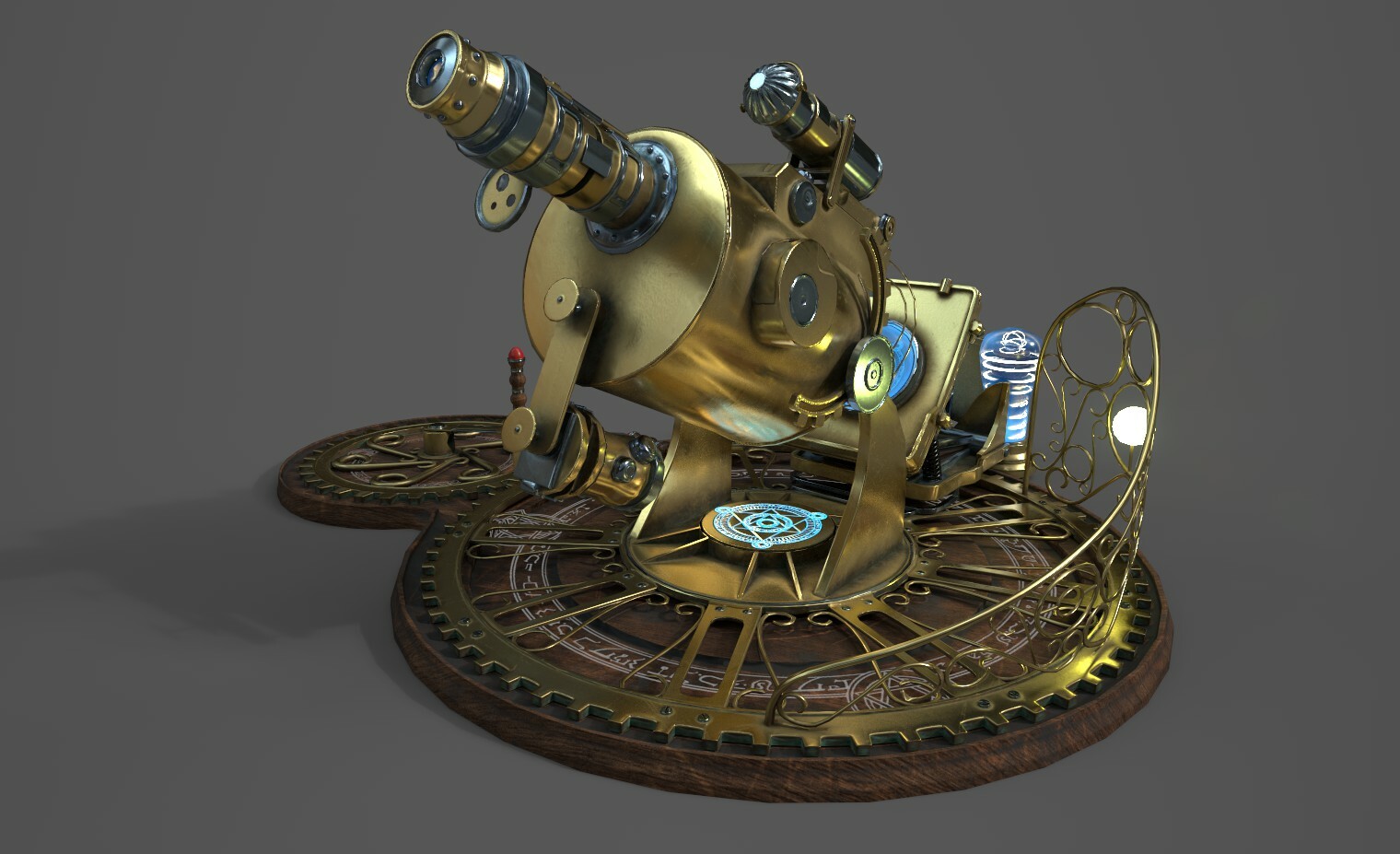This detailed image showcases a steampunk device that blends functional aesthetics with imaginative design, appearing to emerge from a video game or animated fantasy. It presents a golden, brass-coated contraption with intricate gears adorning its base, suggesting the appearance of a vintage microscope or a metallic, cylindrical cannon. The device features multiple cylindrical eyepieces with gold and blue accents, extending from a central tube-like structure that might be seen in compression devices or fishing reels.

The apparatus rests on a wooden base with brass and metallic embellishments, including curved, fence-like extensions. The center and left sides reveal circular components, some with rotating sections and clock-like faces, emphasizing the intricate mechanical craftsmanship. A small, flashlight-like light is inserted into the left corner, pointing upwards, while a round, illuminated area is visible on the center right. Additionally, a light blue, possibly neon light, glows in the background over a dark grey backdrop.

Overall, the horizontally rectangular image, clearly lit with artificial light, presents a striking blend of steampunk aesthetics with metallic brass, clockwork gears, and blue accents, creating a bizarre yet captivating mechanical masterpiece.